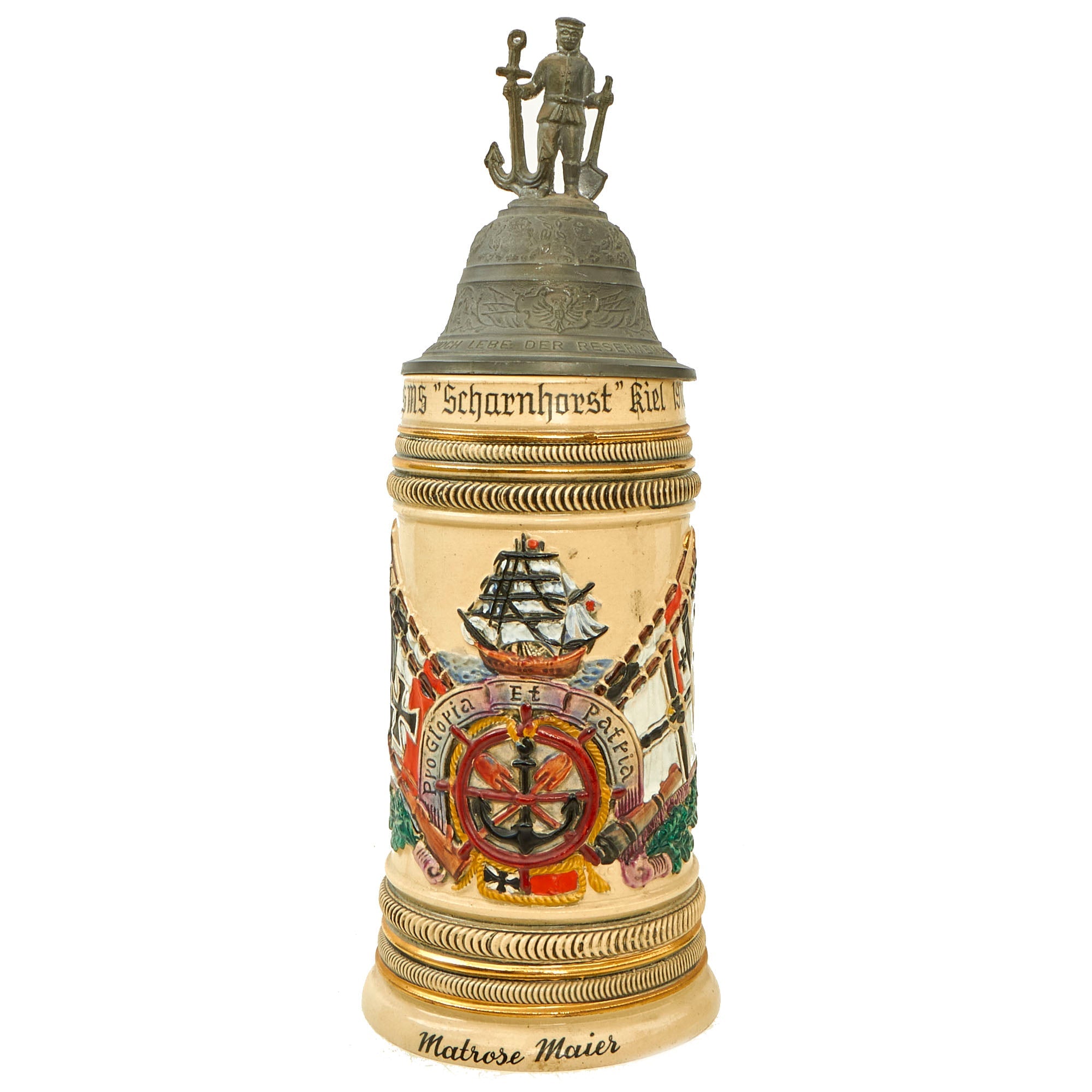The image features a largely metallic bell that exhibits a notable antique and vintage aesthetic. At its pinnacle stands a small, intricately detailed statue of a man, who holds a shovel in one hand and an anchor in the other, symbolizing a maritime theme. The upper section of the bell is dark grey, adding a rustic allure, while the lower portion is brightly colored, predominantly green with a vibrant and intricate design. This design showcases maritime symbols, including a ship and sailor insignia, reflecting its nautical inspiration. Notably, at the base of the bell, the name "Matt Rose, Mayor" is inscribed in black. The background of the image is stark white, which accentuates the detailed craftsmanship and historical charm of the bell.